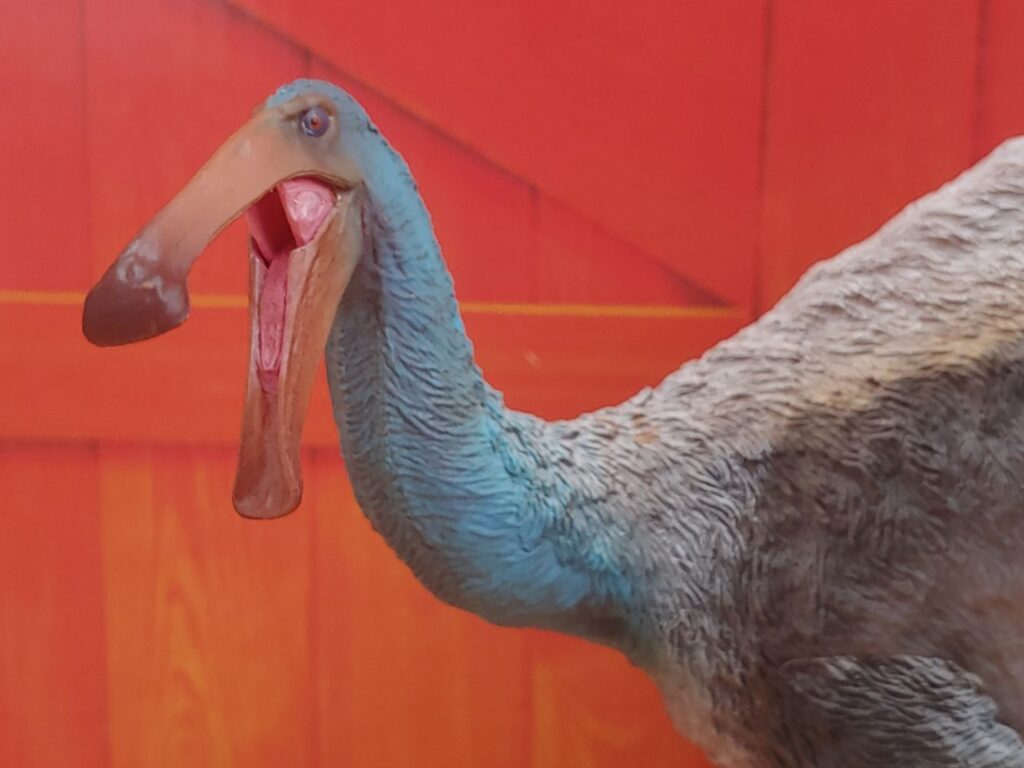The image features a detailed sculpture of a bird-like creature, which exhibits several unique characteristics. The bird is viewed from a side angle, with its head slightly tilted towards the viewer, revealing an open beak that displays a pink interior and tongue. The extensive beak is light brown with a darker tip. Covering its seemingly large and humped body, the sculpture has meticulously carved gray feathers, mimicking the texture of fur. The bird’s long neck is slightly curved and appears bluish in hue, while its eyes, seemingly angry, have small red centers. The sculpture bears a striking resemblance to an ostrich but with a distinct, elongated, dinosaur-like demeanor. The backdrop consists of a vibrant wooden barn door, displaying shades of red, orange, yellow, and brown, adding to the overall rustic and vivid atmosphere of the setting.